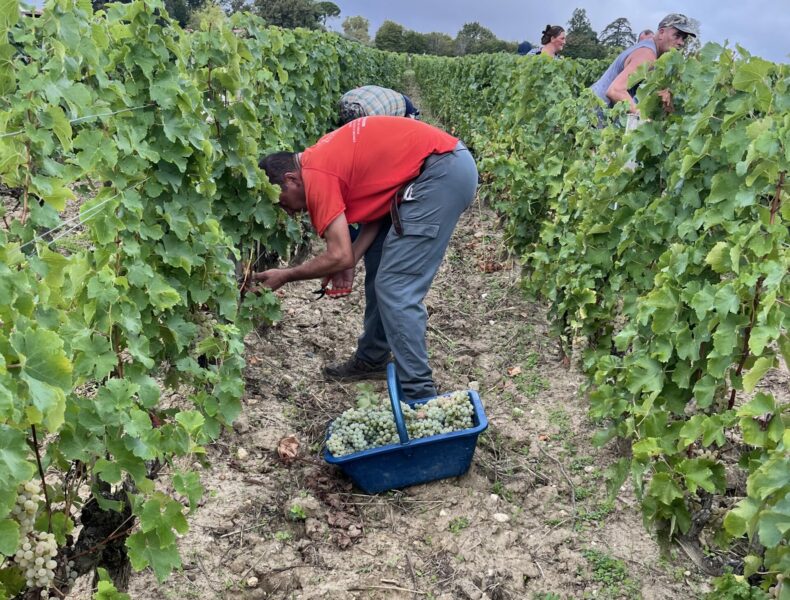This detailed color photograph captures a busy vineyard harvest in a rectangular frame that is wider than it is tall. The ground, a rich brown dirt, is dotted with rows of lush grapevines laden with small green grapes. A large blue bin overflowing with freshly picked grapes dominates the scene.

In the foreground, a man in a red t-shirt and gray, cargo-style pants, with tan arms, is bent over, diligently picking grapes from the vines. His sneakers show signs of a hardworking day in the field. Just behind him, a woman in a white and blue checkered shirt and blue pants is similarly engaged in harvesting, her hair neatly tied up in a bun. Further back, to the right, another worker in a blue tank top and camouflage hat continues the task, illustrating the collaborative nature of the vineyard's workforce.

The background reveals more rows of grapevines and additional workers, what appears to be a total of five people, all focused on the harvest under an expansive blue sky. This picturesque vineyard scene showcases the dedication of the laborers amidst the serene and orderly rows of grape plants.